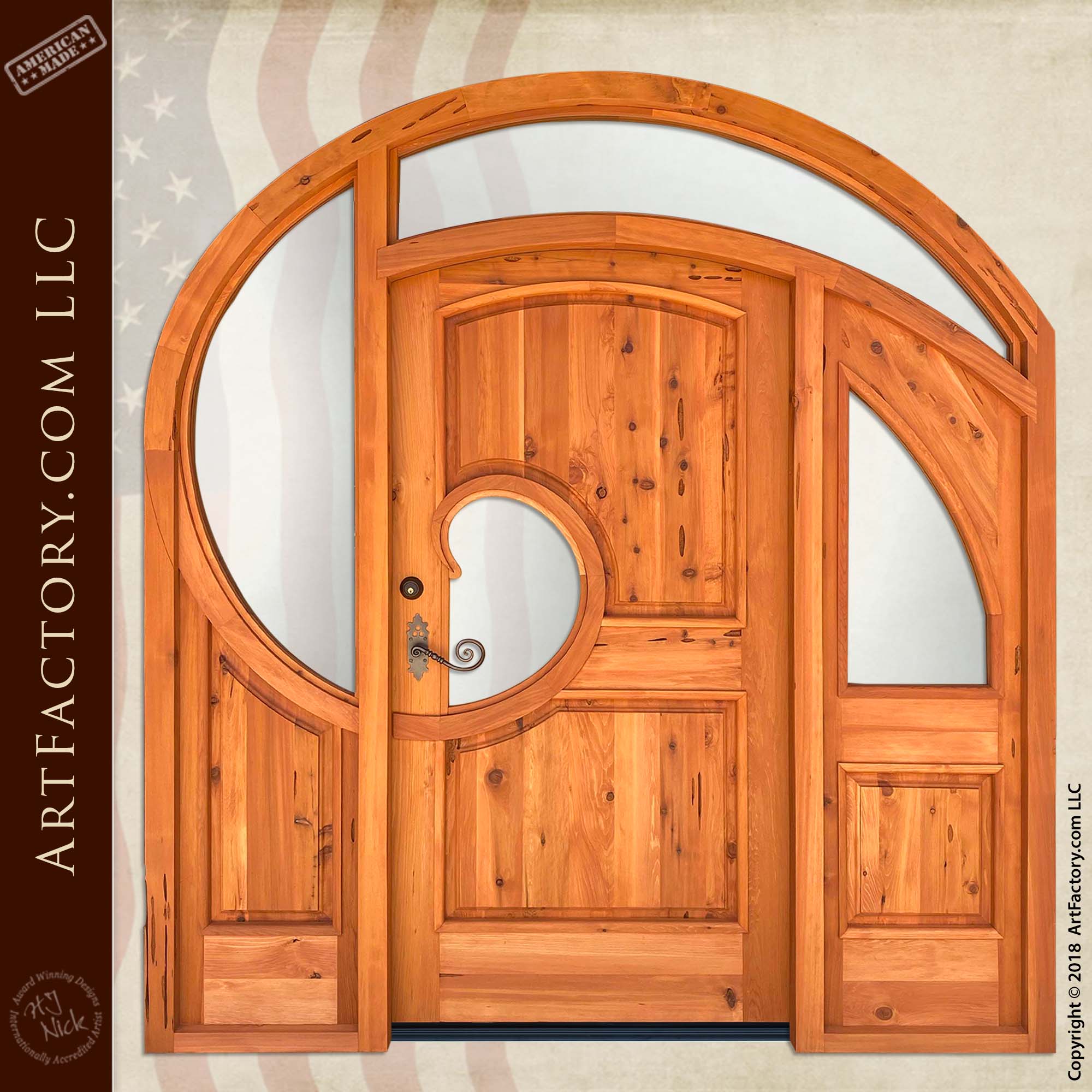The image depicts a large, ornate door crafted from wood with a light brown to light redwood hue. The door features a significant amount of intricate, swirling wooden designs, including a swirl motif present in the door panels and the doorknob, which is also black with a delicate swirl at its end. The door also incorporates glass elements, artfully arranged to form elegant, curving patterns, enhancing its innovative and unique appearance. Additional details on the door include a black keyhole and three notable inscriptions: on the top left, “American Made”; on the left side, “artfactory.com, LLC”; and on the bottom right, “© 2018 artfactory.com, LLC.” In the background, part of an American flag in red, white, and blue is visible, adding a contextual backdrop to the image.